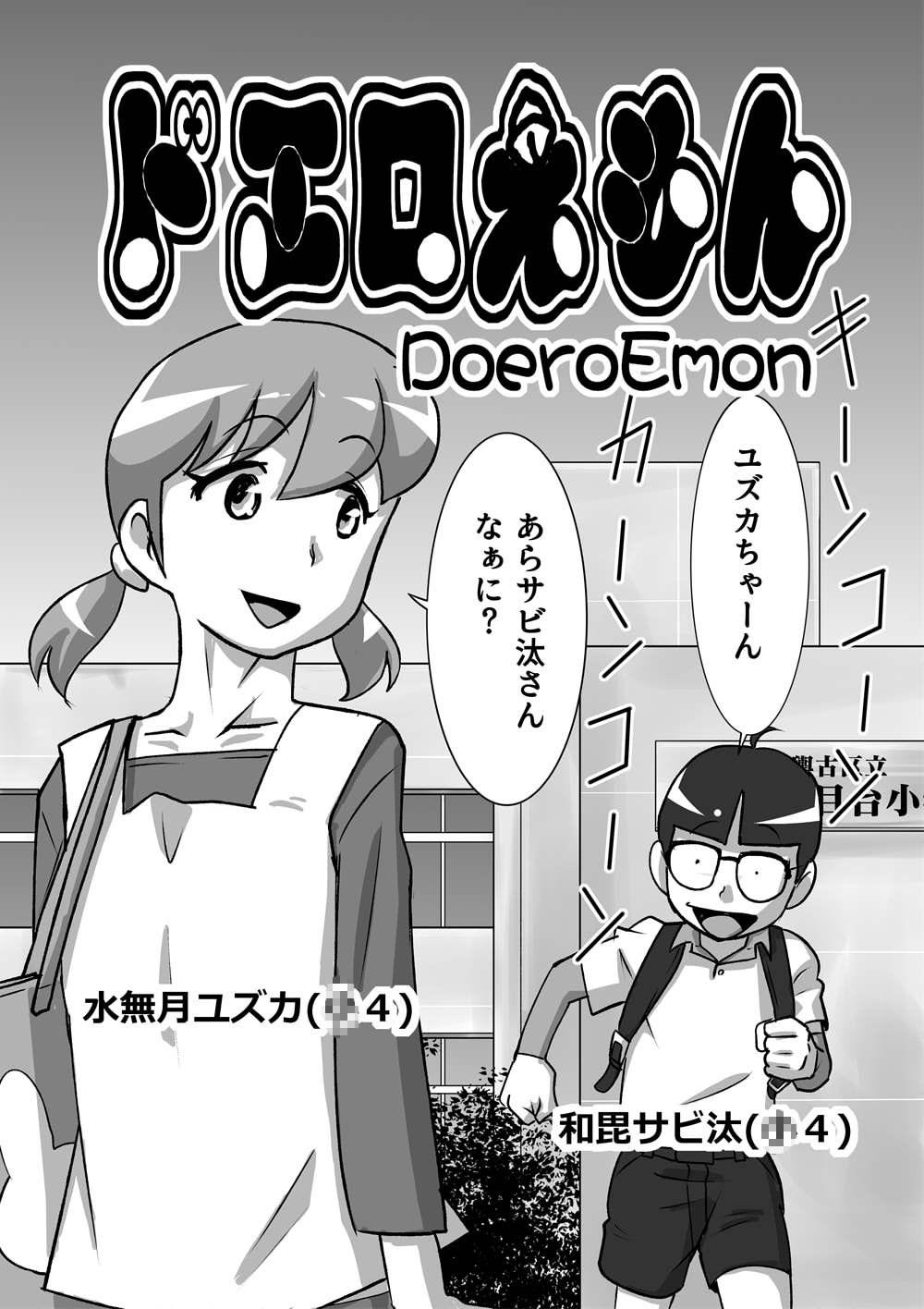The image appears to be the cover of a Japanese comic book. It features a detailed black-and-white illustration, dominated by shades of gray. At the top of the cover, there are lines of black Japanese text with white borders, presumably the title and other information. Underneath the Japanese text, the English words "Doerman" are prominently displayed.

In the central part of the image, a young girl and boy are depicted standing in front of a square, two-story building composed of various gray squares with windows on the left side. A shadow of a leafy bush is cast on part of the building, adding depth to the scene.

The girl is positioned on the left. She has pigtail-styled hair and wears a white smock over a long-sleeve shirt, carrying a purse on her shoulder. She is looking back toward the boy with her mouth open, suggesting she is speaking, although her speech bubble contains Japanese text. 

The boy, slightly behind her to the right, has short dark hair and is depicted wearing a light short-sleeve polo shirt, dark shorts, gloves, large glasses, and a backpack. He appears animated, smiling with his tongue out, and is running towards the girl. Both characters have additional Japanese text positioned around their stomachs, each featuring a parenthesis with the number 4. 

Overall, the intricate linework and interplay between the black, white, and gray tones give the cover a striking, classic comic book aesthetic.